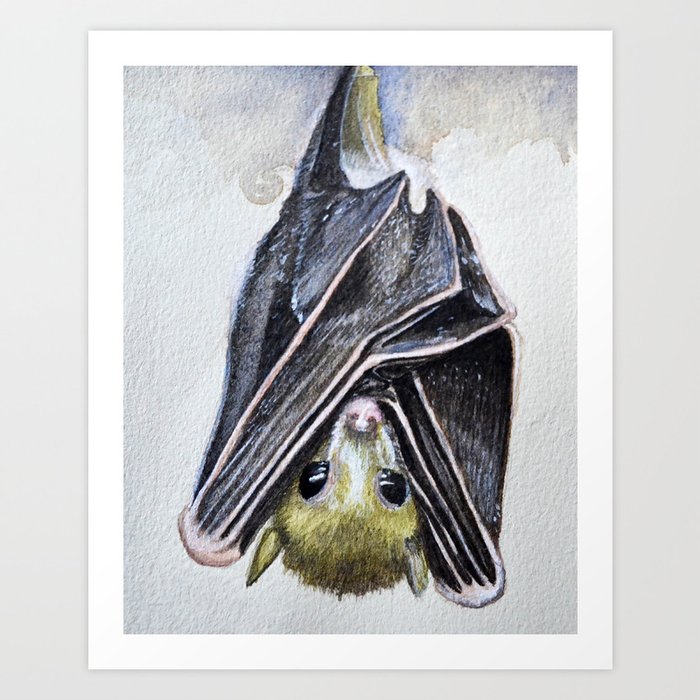This vertically rectangular artistic print features a detailed sketch of a bat hanging upside down against a smooth, gray background. The bat, drawn with a mix of watercolor textures, has a striking appearance with its large, black beady eyes that reflect light, a pink nose, and brown fur around its head. Its ears are pointed downwards, and its delicate, folded wings display black and white stripes with pink edges. At the top of the bat, there is a small green section blending into a gray and blue upper background, creating a stark contrast. The piece is framed by a subtle white border, adding a clean finish to the rough, artistic rendering of the bat’s natural elegance.